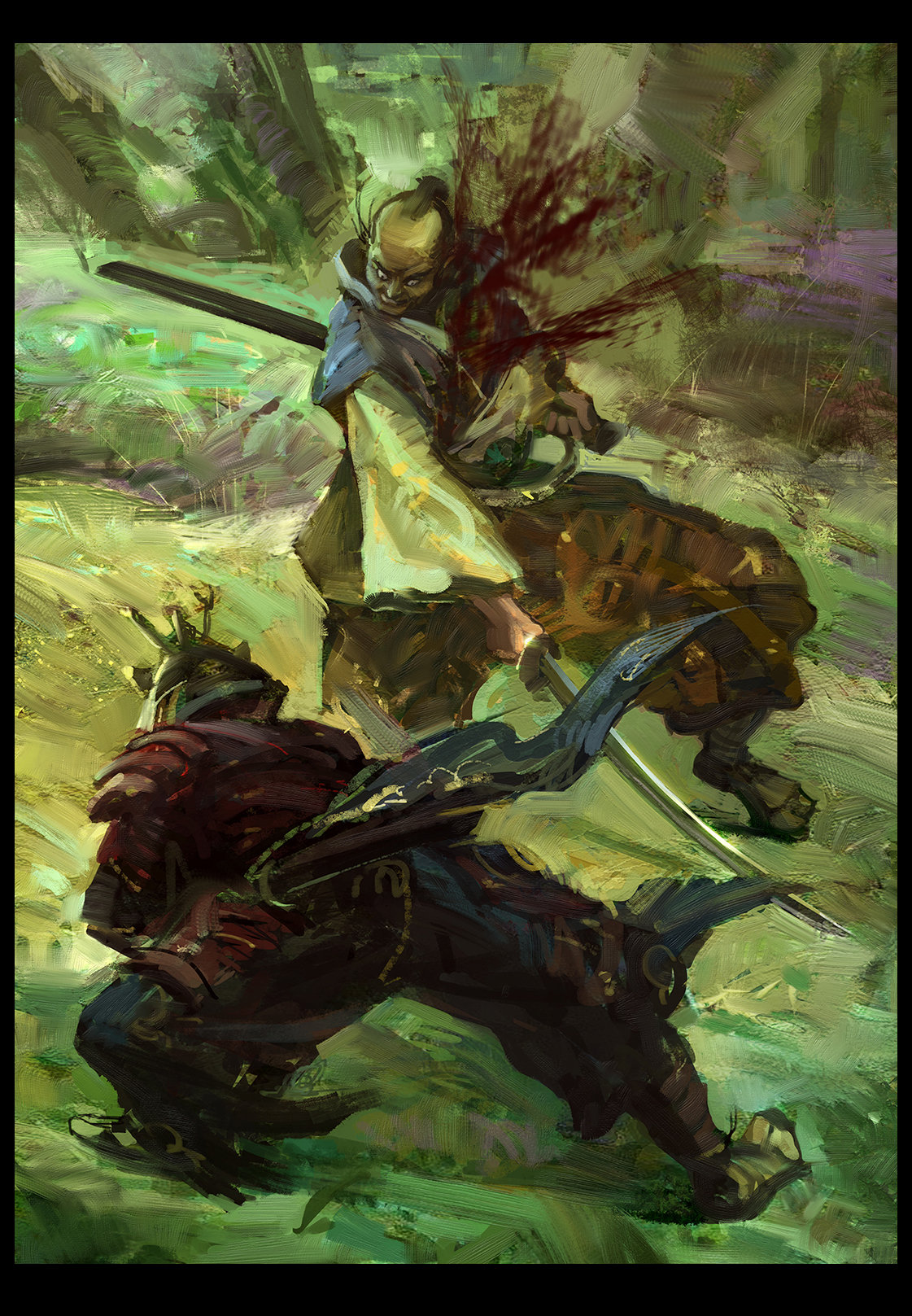This vivid oil painting depicts an intense battle between two samurais set against a lush forest backdrop. The ground, painted in vibrant shades of green, suggests grass, while a towering brown tree enveloped by large green leaves occupies the top left corner. A surreal, purplish lake peeks from the top right corner, adding to the otherworldly atmosphere.

The samurai in the background is a bald ronin with a long, black ponytail. He wears a traditional samurai outfit comprising a blue vest, an underlying white shirt, brownish pants, and sandals. His face, marked by a surprised expression, has wide-open eyes and mouth. He grasps a katana with his right hand, which is slashed downward, while the sheath dangles from his left side. Blood gushes from the left side of his chest, captured in striking red paint strokes.

In the foreground, closer to the viewer, is the second samurai with his back turned. He is slightly bent over, seemingly dodging an attack. This warrior wears a dark red vest, blue pants, and a silver cone-shaped helmet adorned with spikes. His feet are clad in sandals, and although his face is not clearly visible, his traditional attire and posture suggest readiness. 

This detailed image combines elements of cultural authenticity with surreal abstraction, portraying a dramatic and dynamic clash between these two warriors.